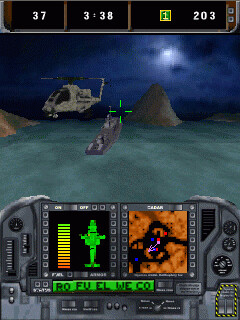This detailed screenshot from a computer game captures a rich, immersive scene featuring a nighttime operation. At the top of the display, there's a scoreboard showing numbers: "37," "3.38," and "1" followed by "2.03," possibly indicating points, time, and status. The main screen provides a cockpit view from a helicopter, complete with flight monitor displays and green crosshairs for targeting. Below, a pixelated warship navigates pixelated blue waters surrounded by islands, with a massive rock prominently positioned next to the ship. The dark sky overhead reveals a moon, suggesting an evening setting. A control panel with various buttons, dials, and an on/off switch is visible, enhancing the immersive gameplay experience.